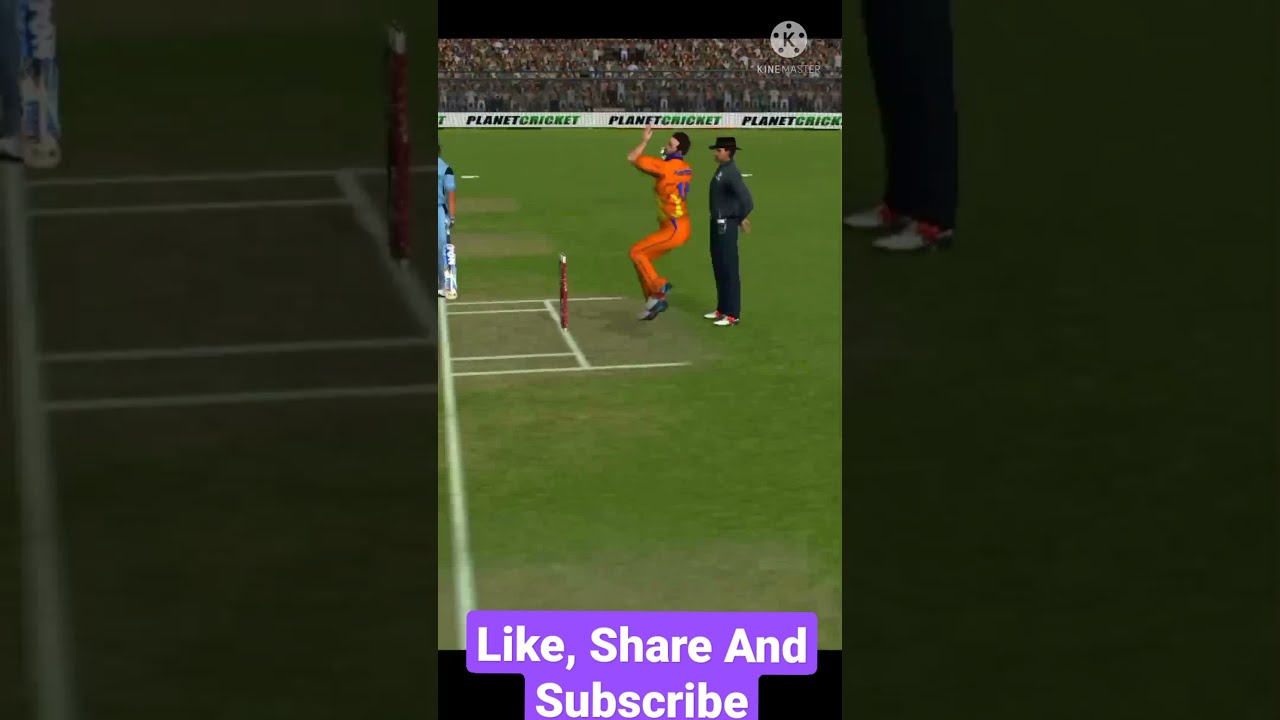This horizontal rectangular image is a detailed screenshot from a video cricket game. At the center, a character dressed in an orange uniform with blue numbers and yellow accents is captured in midair, seemingly in the act of pitching a ball. Positioned behind him, a figure adorned in a black hat, black shirt, and pants, and distinctive white and orange saddle shoes stands ready on the grass. The dynamic visuals are framed with a black border on both the top and bottom edges. Below, white letters on a purple background encourage viewers to "Like, Share, and Subscribe." The background reveals a lush green field with a crowd-filled stadium visible at the top. The banner displaying "Planet Cricket" (with "Planet" in black and "Cricket" in green) stretches across the seating area. The field's boundaries are accentuated by white chalk lines and a red stake with a white tip on the left. Vertical rectangles on either side of the main image fragment the scene with close-ups of the field—on the left, a tight view of white lines, and on the right, a partial view of the character in black. This comprehensive layout immerses the viewer in the vibrant cricket game, blending live action with a call to engagement.